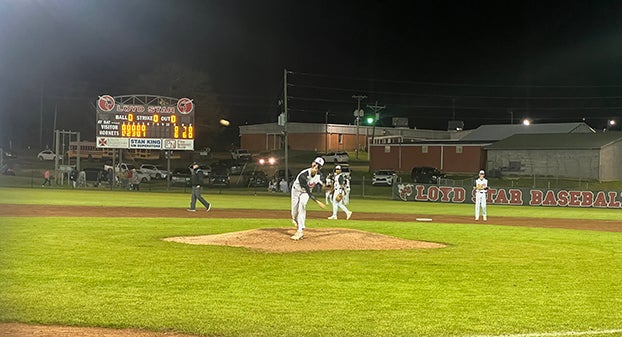The photograph captures a high school night baseball game at a professional stadium, featuring a pitcher in mid-throw on the elevated dirt pitcher's mound. The umpire is positioned between second and third base, while the second baseman, shortstop, and outfielders are also visible. The scoreboard, casting a bright light, hints at the name "Floyd Star Baseball" and possibly "Hornets" leading 6-0. A residential area with parked cars and school buildings frames the background, with additional players and spectators milling about in the left field. The game appears to be in the 5th inning, under a black sky illuminated by the stadium lights.